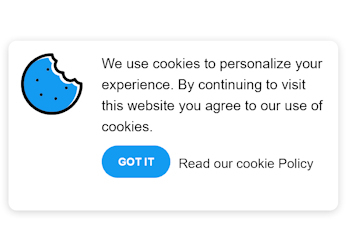The image features a pop-up notification from a webpage, clearly set against a white background. This pop-up is rectangular with rounded edges and is approximately twice as long as it is tall. The outer border of the rectangle is gray, while the interior is white, providing a clean and simple aesthetic.

In the right center of the pop-up, there is a message in black text that reads, "We use cookies to personalize your experience. By continuing to visit this website, you agree to use our cookies." Directly below this message, there is a clickable blue oval button with white text that says, "Got It". Additionally, beneath the button, there is a link in black font that says "Read Our Cookie Policy".

At the top center of the pop-up, there is a logo or image of a partially eaten cookie. This cookie has a black outline and black dots, likely representing chocolate chips, with a blue interior. This playful graphic leverages the dual meanings of the word "cookie" to create a humorous and approachable element in the notice.

The entire scene is devoid of any other website identifiers or additional context, leaving the focus solely on the cookie usage notification.